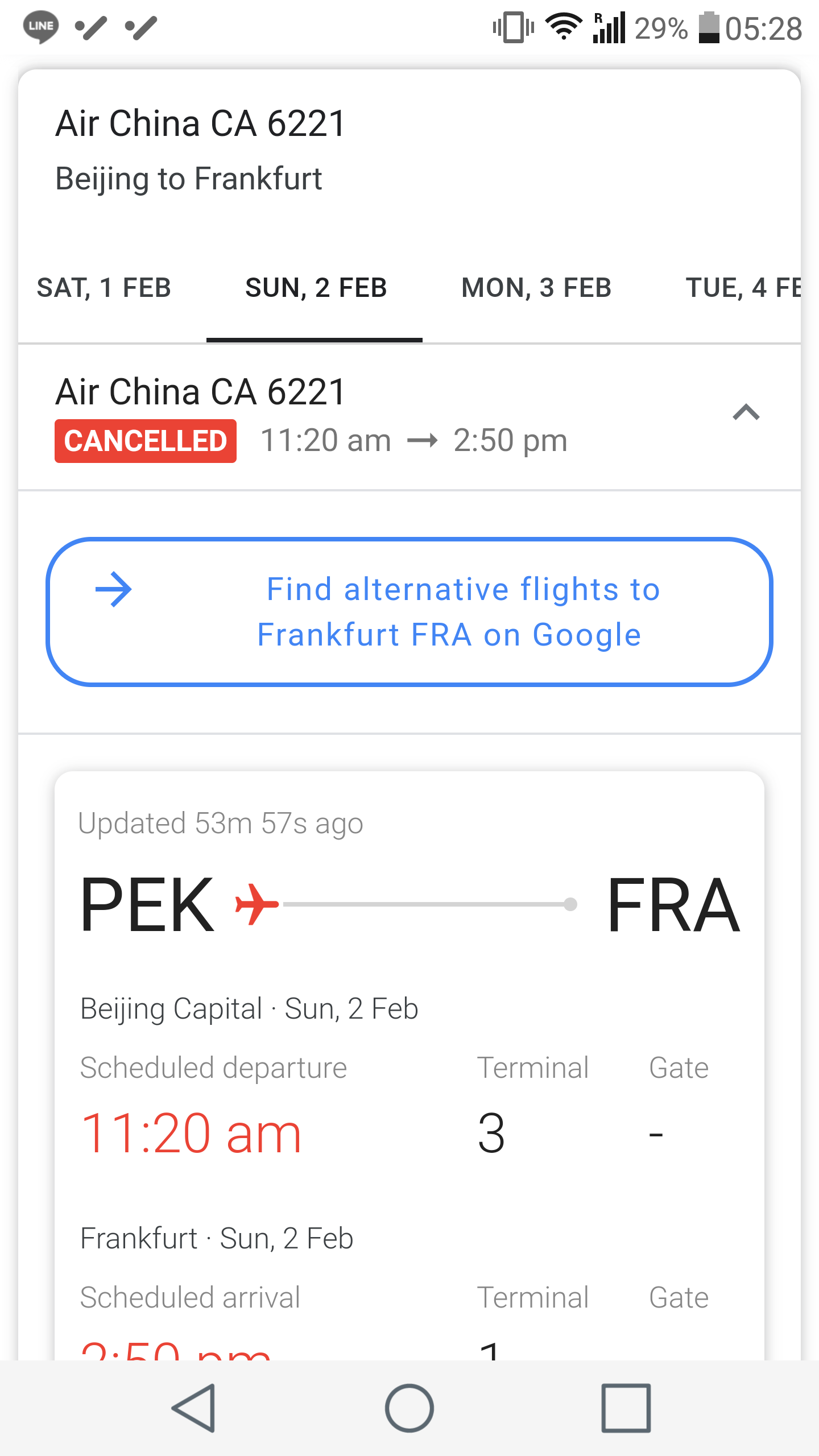The top left corner displays a series of icons: a speech bubble, two dots with a slash in between, a vibrating phone, and a filled Wi-Fi signal. Below these, signal bars show 29%, and the time is indicated as 05:28.

The image also features multiple text elements:

- Locations: Texas, Air, China, California, Beijing, Frankfurt.
- Dates: Saturday, 1st February; Sunday, 2nd February; Monday, 3rd February; Tuesday, 4th February.

A red rectangle with the word "Cancel" is prominently shown alongside the flight number Air China 6221. The scheduled time 11:20 a.m. - 2:50 p.m. is listed beneath it.

A blue oval suggests finding an alternative flight to Frankfurt (FRA) through Google. An update timestamp indicates that the information was last updated 53 minutes and 57 seconds ago.

Further details include a mention of P.E.K., a red airplane icon, and the route from Beijing Capital Airport (PEK) to Frankfurt (FRA) on Sunday, 2nd February. The scheduled departure time is 11:20 a.m., and the terminal and gate are referenced as Terminal 3.

The bottom section also notes that the flight Air China 6221 was canceled. Additionally, there are directional icons including a left arrow, a circle, and a square.